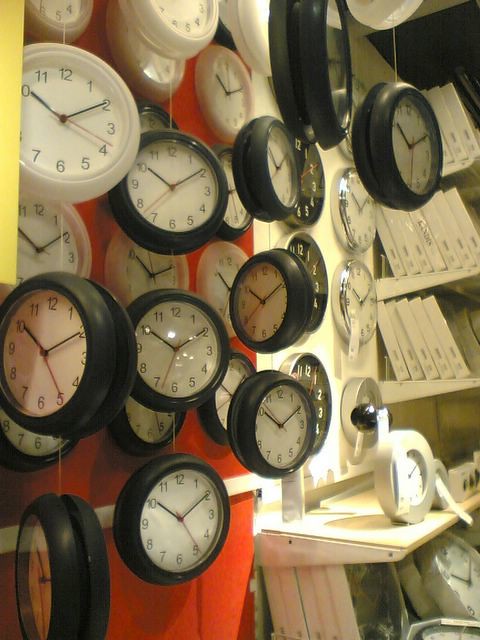This photograph captures an indoor display area filled with numerous circular clocks, predominantly black and white in color. The clocks, all showing approximately 2 o'clock, have white faces with black numbers and black hour and minute hands, along with a red second hand. The backdrop features a wall that transitions from red to white. Some clocks are attached to the red wall while others hang from the ceiling, creating a dense and visually striking effect. Many of these clocks are black-framed, while some are white-framed. Below the hanging clocks, a table draped with a red tablecloth supports additional clocks stacked on top of each other. To the left, an unidentifiable small yellow box is partially cut off from the picture, while to the right, several sealed cardboard boxes with black text are neatly arranged on white shelving. These shelves also hold additional clocks featuring both silver and black frames, adding to the diverse assortment. The setting suggests a retail environment, reminiscent of a store like Ikea, showcasing an elaborate array of timepieces.